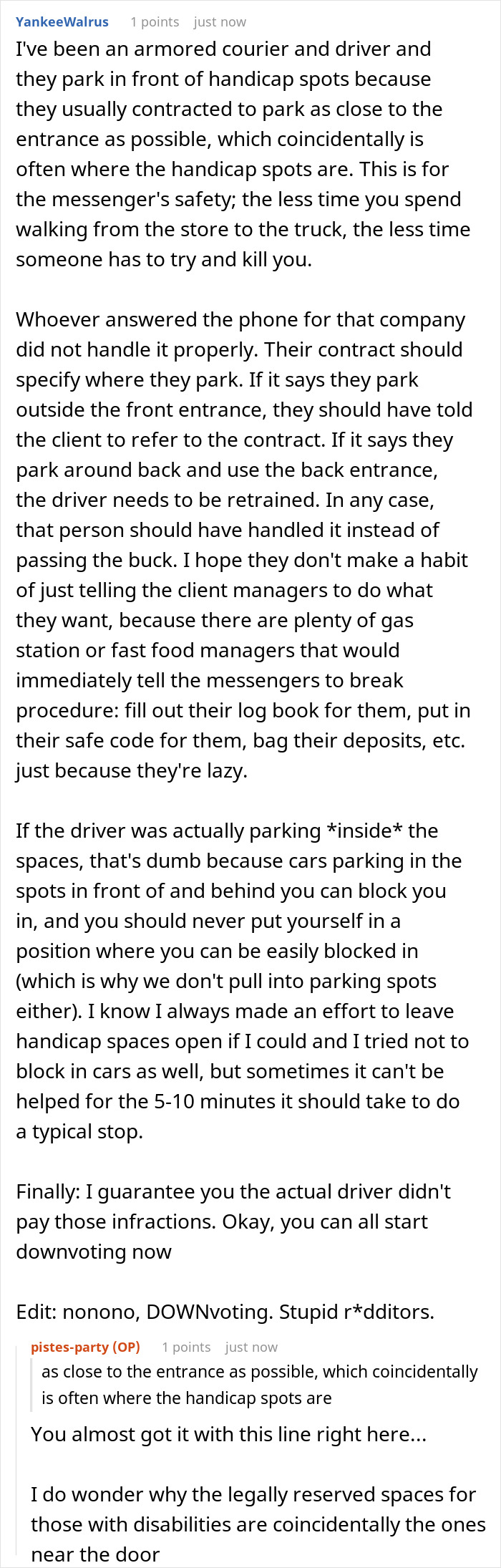The image features a white background with black text and a thin blue line on either side. At the top, in blue text, it states "Yankee Walrus." The text explains the practices and challenges faced by armored couriers and drivers, particularly addressing why they often park in handicapped spots. It mentions that these couriers are usually contracted to park as close to the entrance as possible for safety reasons, as minimizing the distance walked between the store and the truck reduces the risk of attacks. The text criticizes the company's phone handler for not properly addressing clients' concerns regarding parking, emphasizing the need for clear contract specifications and adherence to protocol. It warns against drivers parking inside spaces due to the risk of being blocked in by other vehicles and stresses the importance of not occupying handicapped spots unless absolutely necessary. It suggests that the actual driver likely did not pay any resulting infractions. The caption concludes with a sarcastic remark about receiving downvotes and is followed by two small replies.